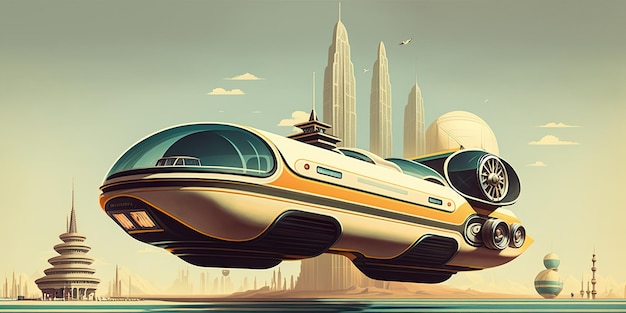The image showcases a detailed, animated depiction of a futuristic, floating vehicle resembling a large bus or submarine, potentially used for public transit. Dominating the center, this sleek, hovering craft features a white body with accents of orange, cream, yellow, and turquoise. It boasts blue windows, gray thrusters, and giant fans at the rear, emphasizing its advanced design. The scene is set against a daytime cityscape with various tall, modern buildings behind it. On the left, there's a unique cylindrical building topped with multiple disks, while on the right, spherical structures with blue lines and spiky, shorter buildings come into view. The bottom of the image has a color textured line in black and turquoise, suggesting it might be floating above an ocean. The sky above is a light blue with a few clouds, enhancing the futuristic ambiance of the scene.